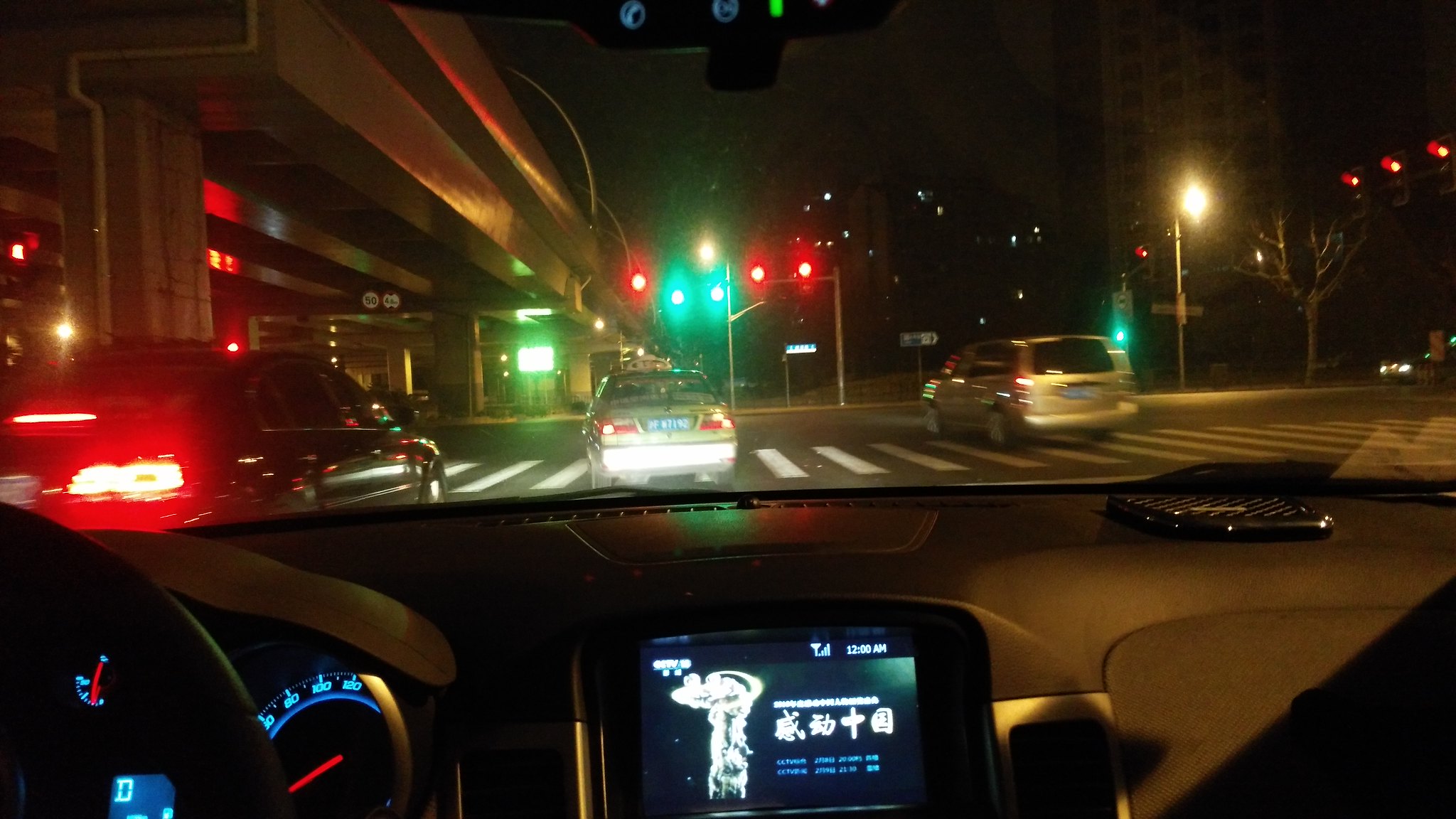A photograph captured from within a car, positioned between the passenger and driver's seats, in an East Asian city. The car's screen prominently displays Chinese characters, indicating its Asian locale, and shows the time as 12 a.m. The scene captures the moment before the car enters an intersection. In the foreground, a black car is situated to the front-left, directly ahead is a gray car, and to the right, a gray van is visible. The urban setting, illuminated by streetlights and the glow of surrounding vehicles, highlights the bustling midnight atmosphere.